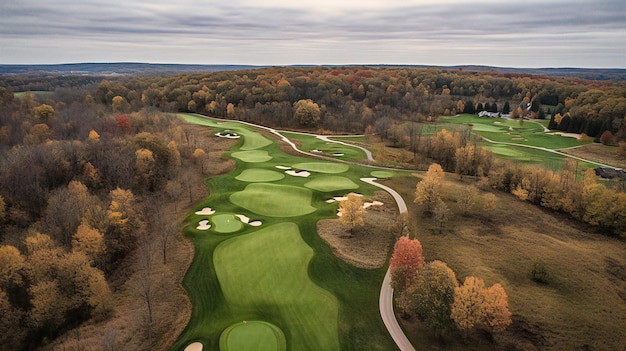This photograph, captured outdoors during the daytime, presents a breathtaking aerial view of a meticulously maintained golf course, possibly taken by a drone. The rectangular image, approximately five inches wide by two inches tall, showcases a complex and beautifully designed fairway set against a backdrop of light gray skies streaked with thin, darker clouds. 

In the far background, low-lying hills are subtly visible beneath the expansive sky. Dominating the center and extending toward the right, the vibrant green grass of the fairway and the greens is interspersed with lighter patches and strategically placed bunkers filled with pale sand. The fairway itself is creatively laid out, segmented into several green islands without flags, suggesting it might be part of a private club given its flawless upkeep.

Paved pathways weave through the course, facilitating easy movement for golf carts. Surrounding the fairway, and particularly prominent to the left, top, and lower right corners of the image, are natural areas dotted with trees in various stages of seasonal change. Some trees are completely bare, while others display a tapestry of yellow and orange leaves, reflecting the autumn setting. This hidden gem of a golf course appears as an oasis within a lush forest, emphasizing its secluded and serene ambiance.